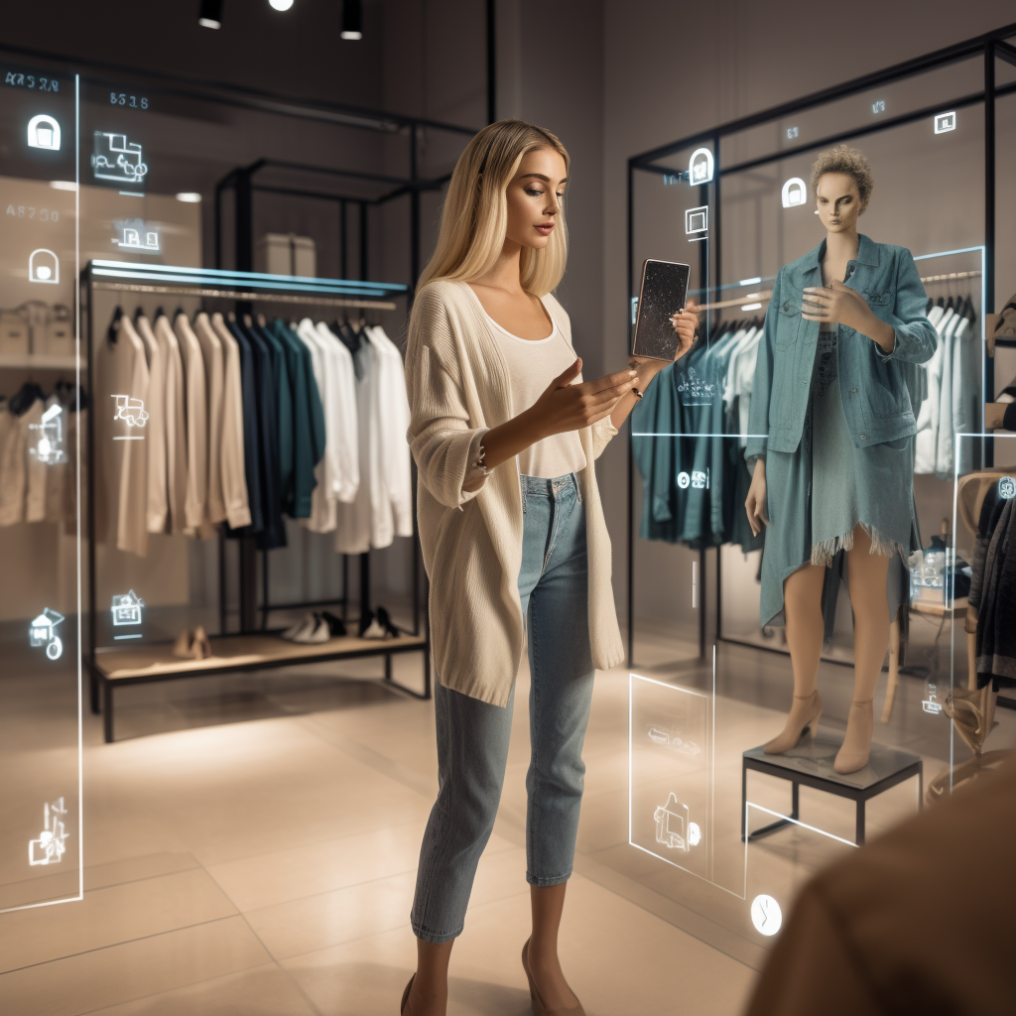In a digital rendering of a futuristic boutique, a blonde woman with shoulder-length hair and brown accents stands at the center, holding a small tablet and gesturing as if conversing with someone on the screen. She has olive skin, pink lipstick, and wears a beige long-sleeved cardigan over a white top, paired with light wash blue jeans cropped at the ankles, and brown heels. The background reveals a sophisticated interior with white walls, digital screens, and hints of smart lens technology. To her right, a mannequin displays a denim jacket and skirt, with beige heels. A clothing rack behind her showcases a gradient of garments: beige shirts to dark blue and white, accompanied by black and white shoes. The floor beneath her is a light beige-brown, complementing the store’s overall modern aesthetic.